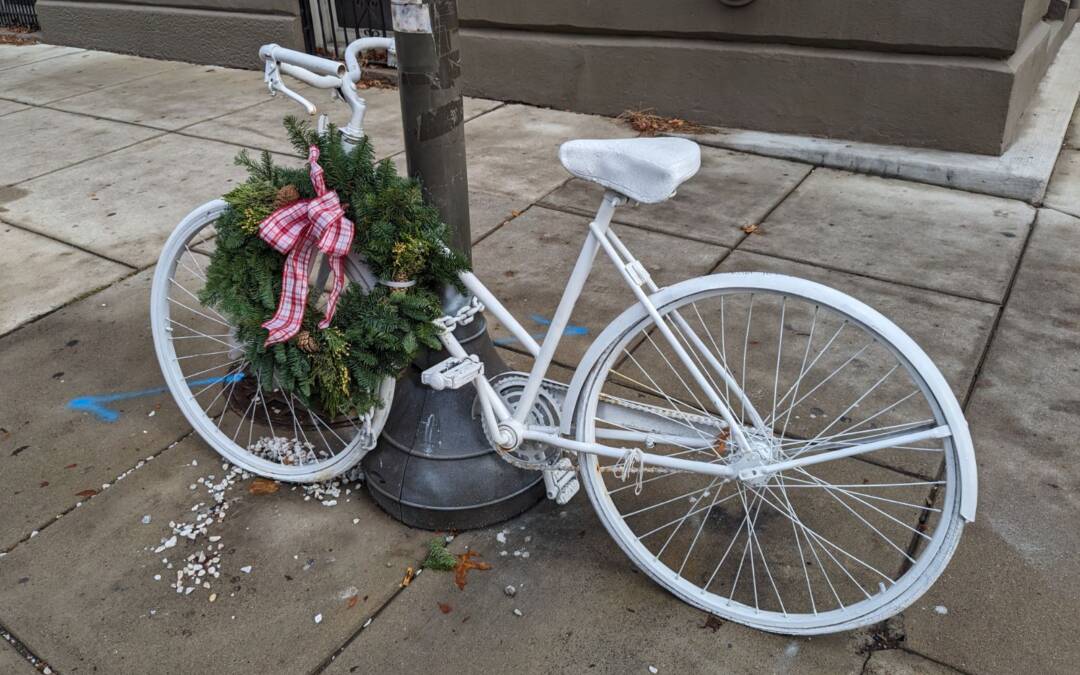In the image, a ghost bike, fully painted white in tribute to a bicyclist killed by an accident, stands chained to a street post. The bike, classic in style, is uniformly white—from the seat and the tires to the spokes and pedals. Even the chain securing it to the post is painted white. The setting is a concrete sidewalk, divided into squares, adjacent to a brownish-gray building corner. A festive wreath of pine needles adorned with a red and white patterned bow decorates the front wheel, signaling a holiday time. The grey and off-white pavement beneath reveals some scattered debris, framing the ghost bike in the center of the scene.